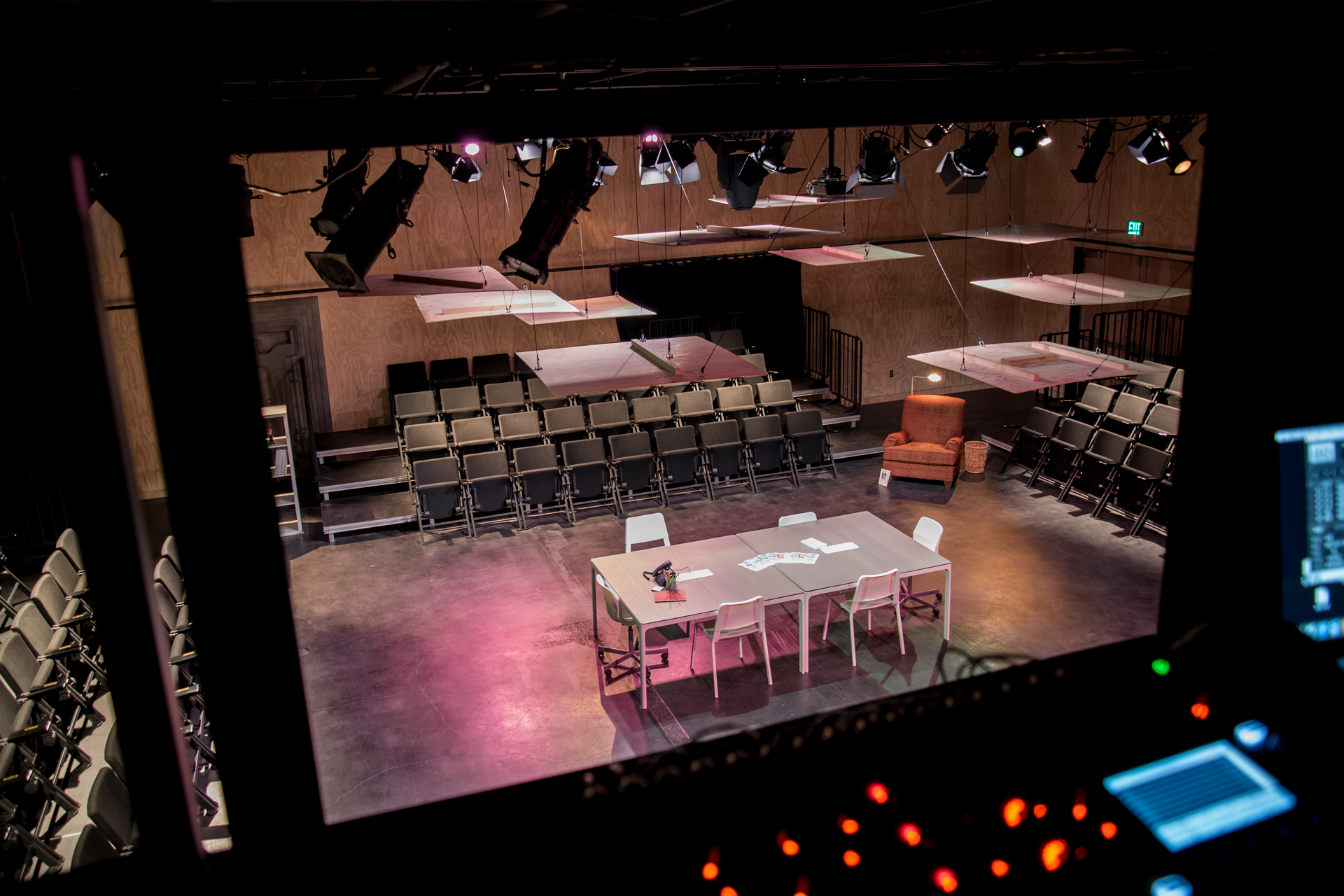This color photograph, taken from an elevated perspective, appears to capture a recording studio or stage setup viewed through the window of a control booth. In the foreground, the control booth houses various blue and white screens with text displays and a complex control panel adorned with red, green, and blue lights. Below the window, the stage features a centrally placed table surrounded by five chairs, with some papers scattered on top. The stage is illuminated by numerous magenta and light orange spotlights suspended from the ceiling. The seating arrangement is extensive, with four rows of empty chairs spanning all four sides of the stage, resembling an auditorium awaiting an audience. The room's walls appear to be wooden, adding a warm texture to the setting. An inviting recliner, paired with a glowing light, is positioned in the upper right corner of the room, suggesting a space for a more relaxed observer. The ambiance suggests a venue primed for performance or recording, though presently vacant.